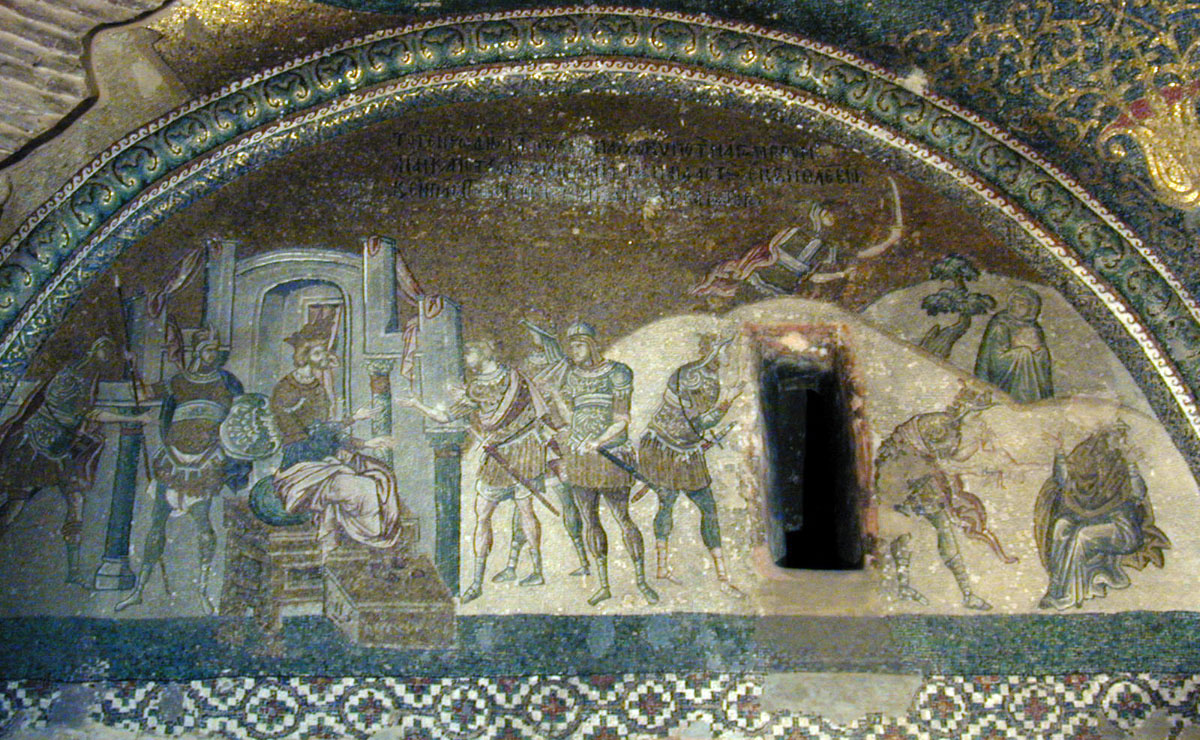The image depicts an elaborate wall painting, likely from a church, which features a partially weathered depiction of historical and possibly religious figures. Central to the artwork is a blue throne with a crowned man sitting upon it, surrounded by what appear to be soldiers, some holding swords while others carry various items such as a basket of fruit. The figures are dressed in robes or armors that suggest a scene possibly from around the 1200s. An ornate archway, adorned with intricate patterns of blues, golds, and whites, frames the painting. This decorative border includes a crisscrossing pattern and a gold-scaled creature with a red crest on its head against a blue background. Below the throne, there is a depiction that might suggest a nativity scene, with more figures possibly seated or standing, adding to the religious significance of the piece. Notably, there is a rectangular hole in the wall—whether part of the original design or a later modification is unclear—which interrupts the lower portion of the painting, exposing the underlying stone where the paint has worn away. Overall, the painting's grandeur and the faded details hint at its age and the history housed within the walls it adorns.